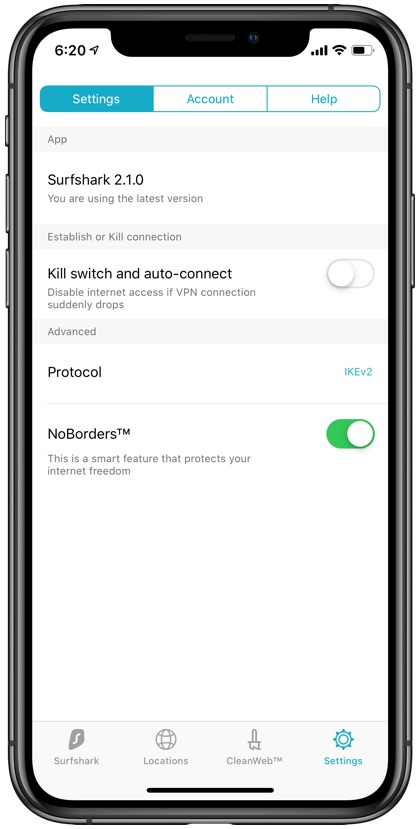This vertical image captures a detailed view of a smartphone screen with a black rim around it. On the upper left corner, the time “6:20” is displayed in black along with a location icon. Across from that, on the upper right, you can see the signal bars, Wi-Fi icon, and battery life indicator. 

To the right side of the phone, various physical buttons are visible, including the power button, volume buttons, and the ringer on/off switch.

The screen of the smartphone is segmented into multiple sections. At the top, a white rectangular strip is divided into three parts: "Settings," highlighted in teal, "Account," and "Help." Below this, in a light gray strip, the version of an application is displayed with the text "Surfshark 2.1.0" in black against a white background, indicating that the user is employing the latest version.

A gray strip reads "Establish or Kill Connection," followed by a bold section titled "Kill Switch" and "Auto Connect," both described as features that disable internet access if the VPN connection drops, with toggles that are currently off. Another gray strip features the word "Advanced," transitioning back to a white background containing "Protocol" in bold black lettering, next to the "IKEv2" option highlighted in teal. This section is separated by a line leading to "No Borders" in black, described as a smart feature that protects internet freedom, with this specific option toggled on.

At the bottom of the screen, there are icons and words for "Surfshark," "Locations," "CleanWeb," and "Settings," with "Settings" highlighted, indicating it is the current selected option.